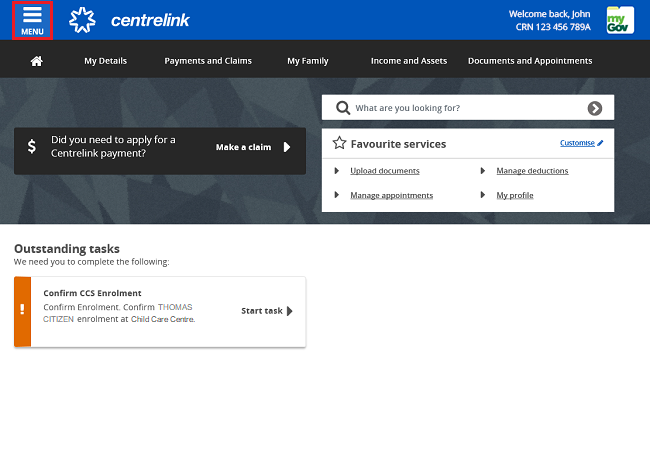This image is a detailed screenshot of a website interface. The top banner is dark blue, featuring white text. On the upper left corner, there's a menu icon enclosed in a red-bordered square. To its right, a star-like logo with the text "In Center Link" is prominently displayed. The upper right corner welcomes the user with the message, "Welcome back John, CRN 123456789A" next to a white square icon labeled "myGov" in green text.

Directly below this is a black, horizontally-aligned banner with white text. On the left side of this banner, there is a home icon followed by various sections: "My Details," "Payments and Claims," "My Family," "Income and Assets," "Documents and Appointments." To the right side of this banner is a search box with a black magnifying glass icon on the left and the placeholder text, "What are you looking for?" A black circle with a right arrow appears on the right side of this search box.

Below this section is another white box. In its upper left corner is a star icon next to the text "Favorite Services," while the upper right corner features the text "Customize" in blue, accompanied by a blue pencil icon. Within this white box are four options listed vertically: "Upload Documents," "Manage Appointments," "Manage Deductions," and "My Profile."